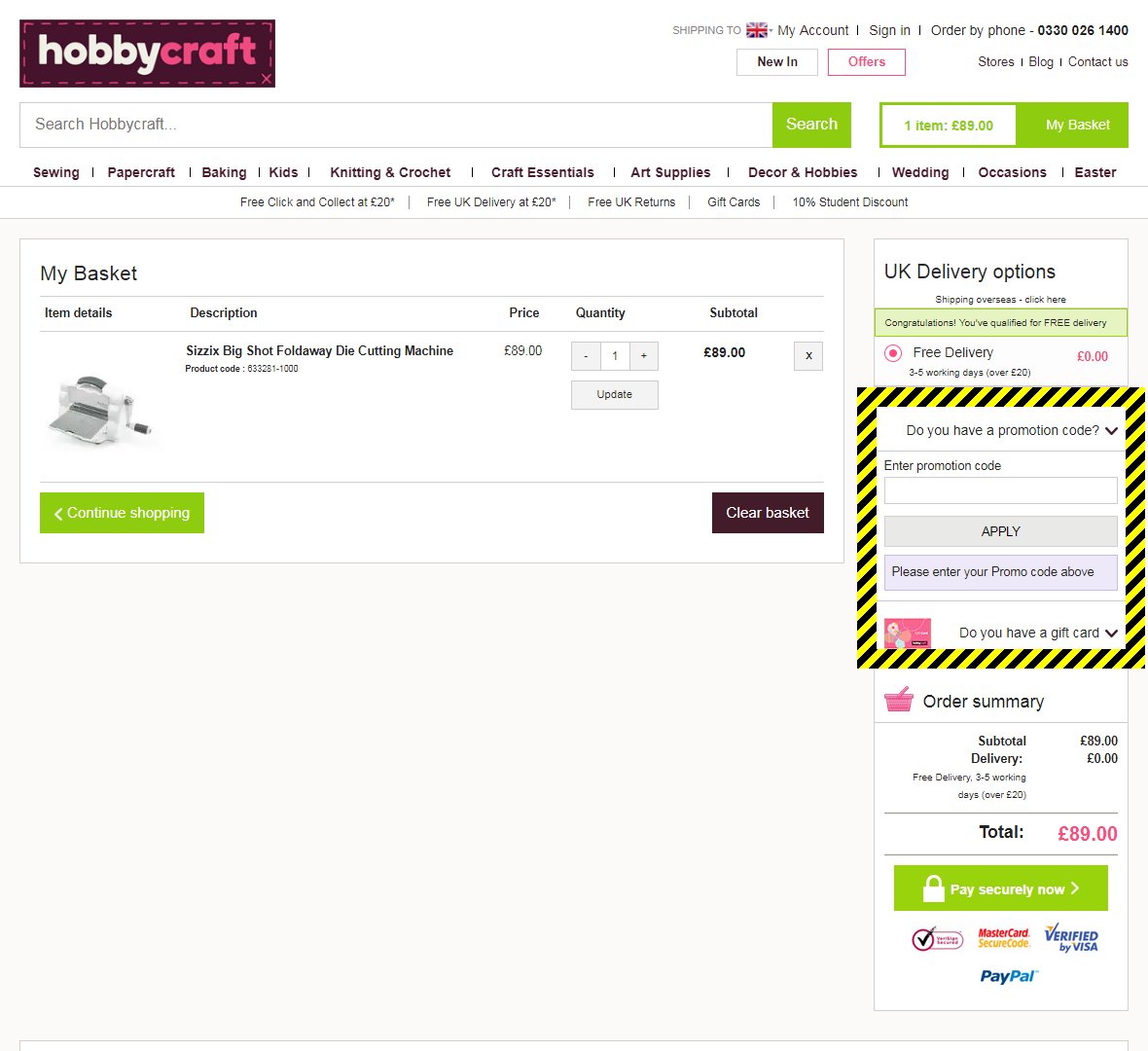**Detailed Caption:**

The screenshot depicts a section of the Hobby Craft website, characterized by a clean white background. At the top, the "Hobby Craft" logo is prominently displayed, with "Hobby" in white and "Craft" in pink inside a striking purple rectangle. Adjacent to the logo are navigation links for "New In," "Offers," "Stores," "Blog," "Contact Us," and options such as "Shipping To," "My Account," "Sign In," and "Order By Phone 0330 026 1400."

Below the navigation bar, there is a handy search bar labeled "Hobby Craft." Next to it, an icon indicates the shopping basket which currently contains one item priced at $89. Additionally, there is a dropdown menu with various categories, including “Sewing,” “Papercraft,” “Baking,” “Kids,” “Knitting & Crochet,” “Craft Essentials,” “Art Supplies,” “Decor & Hobbies,” “Wedding,” “Occasions,” and “Easter.”

A detailed view of the shopping basket is shown on the right side of the screenshot. It includes an itemized list featuring a picture of a sewing machine, its description, the price (specified as $89 or 89 pesos), the quantity (1), and an update option. The subtotal is clearly marked as $89.

At the bottom of the basket interface, there are two prominent buttons: "Continue Shopping" in a green rectangle on the left, and "Clear Basket" in a purple rectangle on the right. Additionally, a note mentions the benefit of "Free Click & Collect" at 20 pesos.